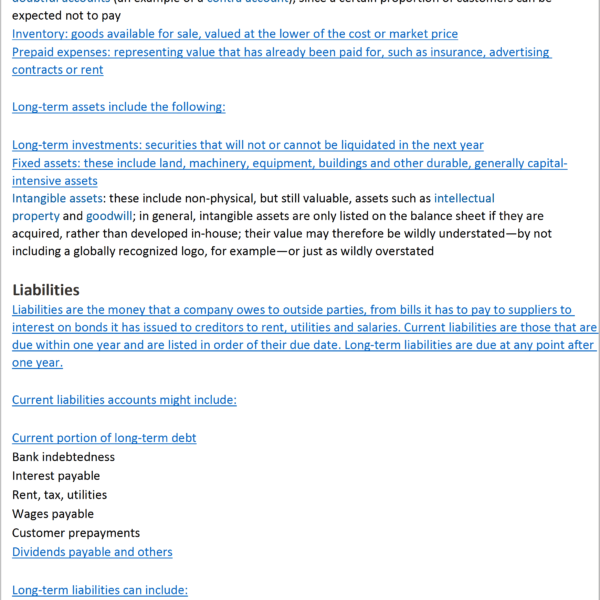The image appears to be a partial screenshot of a web page, most likely from a detailed financial or business document, possibly related to accounting or legal guidance. The top portion of the text is cut off, but it begins with the phrase "expected not to pay." The document outlines various categories of financial information, structured as follows:

- **Inventory**: Goods available for sale, valued at the lower of cost or market price.
- **Prepaid Expenses**: Representing value already paid for, such as insurance, advertising, contracts, or rent.

Following this section, the document discusses long-term assets, including:

- **Long-term Investments**: Securities that will not or cannot be liquidated within the next year.
- **Fixed Assets**: Land, machinery, equipment, buildings, and other durable, capital-intensive assets.
- **Intangible Assets**: These non-physical yet valuable assets encompass intellectual property and goodwill. Importantly, intangible assets typically appear on the balance sheet only if acquired, not developed in-house. This can lead to a significant undervaluation or overvaluation, depending on whether a globally recognized logo, for example, is included or excluded.

The section on liabilities explains:

- **Liabilities**: The money a company owes to external parties, including bills to suppliers, interest on bonds issued to creditors, rent, utilities, and salaries. 
- **Current Liabilities**: Debts due within one year, listed in order of their due dates. Examples include current portions of long-term debt, bank indebtedness, interest payable, rent, tax, utilities, wages payable, customer pre-payments, and dividends payable.
- **Long-term Liabilities**: Obligations due after one year, though the text here is cut off.

Given the detailed and precise nature of the content, it suggests that the source may be a tax, business, or legal advisory website. The visual layout includes a traditional white background with black text and some blue-highlighted sections, though there is no identifiable logo to confirm the exact source of the text.